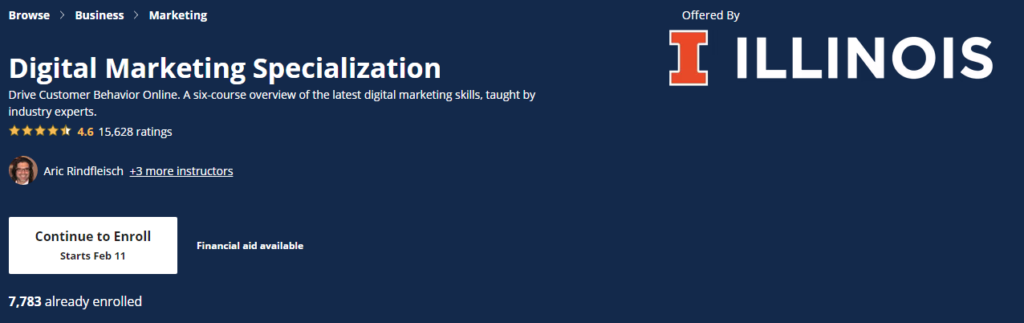Screenshot of a Digital Marketing Class Offered by Illinois

In this web post, a detailed screenshot captures a digital marketing specialization course provided by Illinois. The title prominently features "Illinois" in the top right corner, with the letter "I" displayed in a striking orange color, contrasting against the white letters. The course aims to equip students with contemporary digital marketing skills and is taught by industry experts.

Key details showcased in the screenshot include:
- Course Description: “Drive Customer Behavior Online,” a six-course series covering the latest in digital marketing.
- Instructor: The primary instructor is Eric Reinfeldt, with three additional instructors also contributing to the course.
- Ratings and Reviews: The course boasts a stellar 4.6 out of 5-star rating, based on feedback from 15,628 participants.
- Enrollment Information: A conspicuous white button against the dark blue background invites potential students to "Continue to Enroll." The course starts on February 1st, and it highlights that 7,783 individuals have already enrolled.

Given the high ratings and substantial enrollment numbers, this course appears to be both popular and well-regarded. Despite the strong interest, it seems there are still spots available for new students.